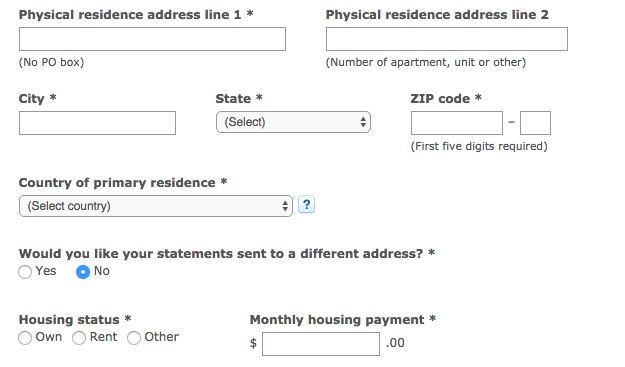The image depicts a form for entering personal information, focusing on residential details:

At the very top left, bold black text indicates "Physical Residence." Below this header are several fields for input. 

1. The first field includes the main address, indicated by an asterisk to the right, signifying it is a required field. This entry box is bold and stands out, but it is currently empty.
2. Underneath, there is a smaller rectangular input box with a placeholder for PO Box entry, which remains empty as indicated by parentheses. It specifies "No PO Box."
3. Another labeled field for specifying "Apartment, Unit, or Other" is present with an empty box at the bottom of the parentheses. 

To the left, the field labeled "City" is in bold black text with an asterisk. The input box beside it remains empty.

Adjacent is a dropdown menu labeled "State," indicated as another required field by an asterisk. No options are currently selected, and the box is described as slightly greyed-out compared to the others. 

To the right, there's a field labeled "Zip Code" with an asterisk. This comprises two empty boxes separated by a dash, the first larger than the second, with a note below in parentheses stating, "First 5 digits required."

Below and to the left, the label "Country of Primary Residence" appears with an asterisk next to it. A dropdown box labeled "Select Country" follows, marked by a blue question mark icon indicating assistance or information is available. It remains unselected.

Further down, a prompt asks, "Would you like your statements sent to a different address?" also marked by an asterisk. The options "Yes" and "No" are provided, with "No" being selected and "Yes" greyed out.

Beneath this, the section "Housing Status" also noted by an asterisk, and input options for "Owner" and "Other" are present, both currently unselected. On the right, there is a field for "Monthly Housing Payment," with an adjacent box for monetary input, currently displaying "$0.00." 

The form requires additional input in several mandatory fields highlighted by asterisks, with placeholders and dropdowns awaiting user selection.